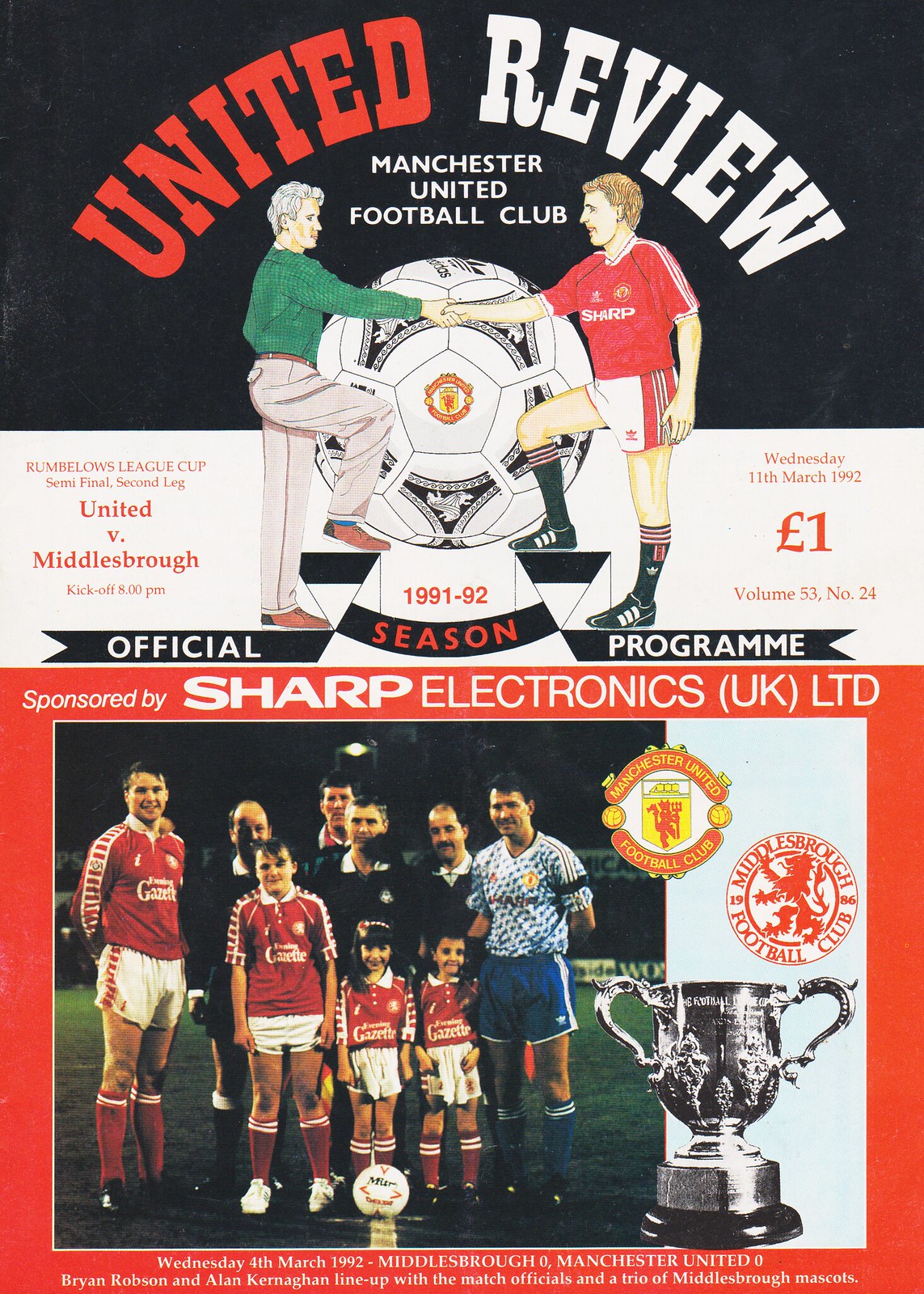On the front page of what appears to be a magazine cover or promotional flyer titled "United Review Manchester United Football Club," two gentlemen are illustrated shaking hands in front of a large soccer ball. Bold red and white lettering prominently displays the title. The left-hand side details "Rumbelows League Cup Semi-Final Second Leg: United versus Middlesbrough," with a kickoff scheduled for 8:00 PM on Wednesday, March 11, 1992. Priced at one pound, this volume is marked as 53, number 24. Sharp Electronics UK Ltd sponsors the publication. Below, there is a photograph of team members wearing soccer jerseys, children supporting the team, and a silver trophy. Additionally, Bryan Robson and Alan Kernaghan are seen with the match officials and Middlesbrough mascots, encapsulating both enthusiasm and anticipation for the match.